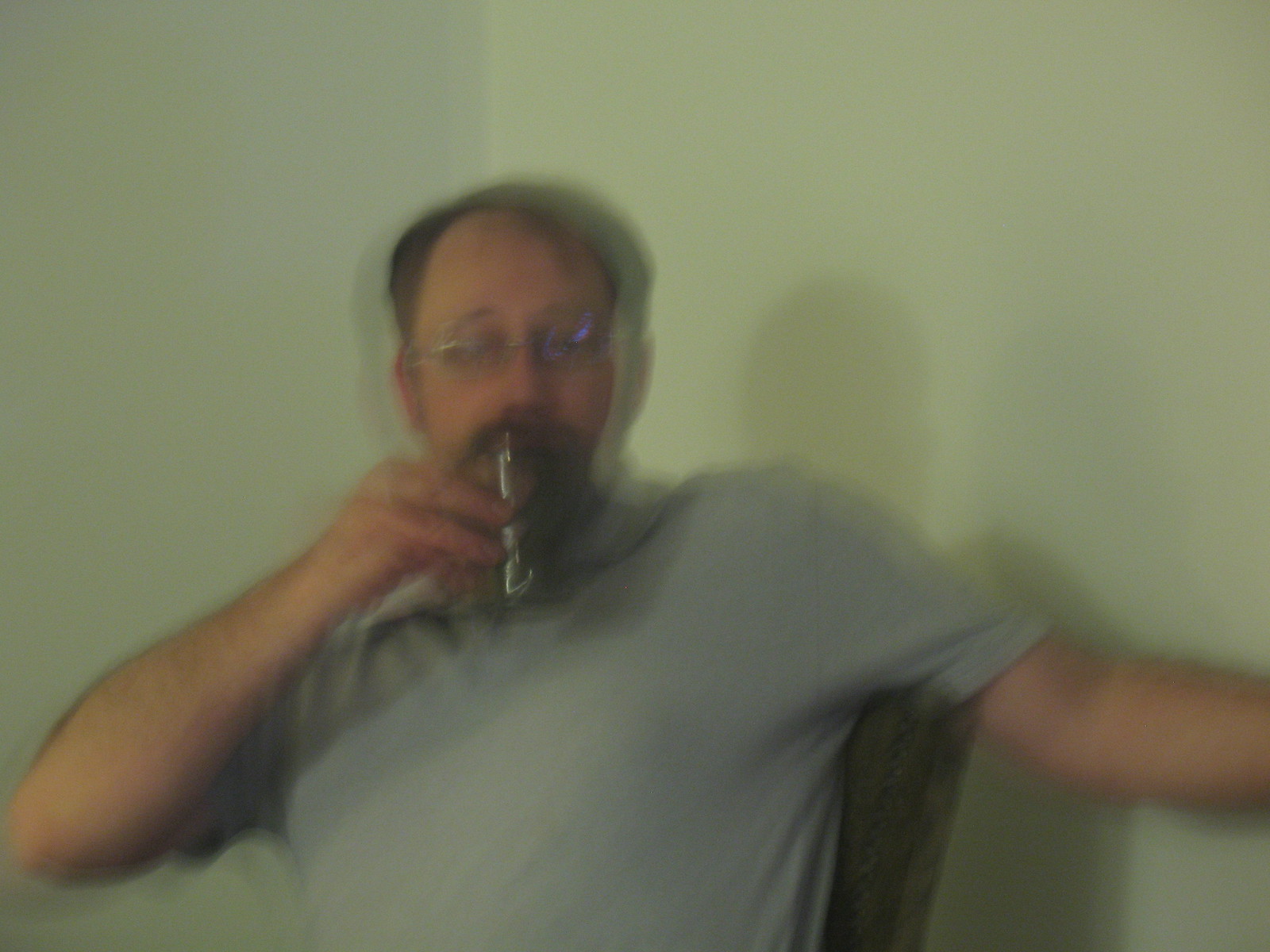In the image, a partially balding, fair-complexioned, middle-aged Caucasian man with medium brown hair, thin silver glasses, a mustache, and a beard, is sitting in a chair positioned in the corner of a room where two light green walls meet. He is wearing a short-sleeved gray T-shirt and gazes directly at the camera. The photo is blurred, adding a sense of mystery. The chair, appearing to be wooden, reveals only a section of its back, and he sits with his left arm extended out of view. His right hand holds an unidentified silver metal object up to his mouth, which could be a pen, a smoking apparatus, or a metal shaver handle with a razor. The image captures him from about the ribcage up, with his shadow faintly visible on the wall behind him.